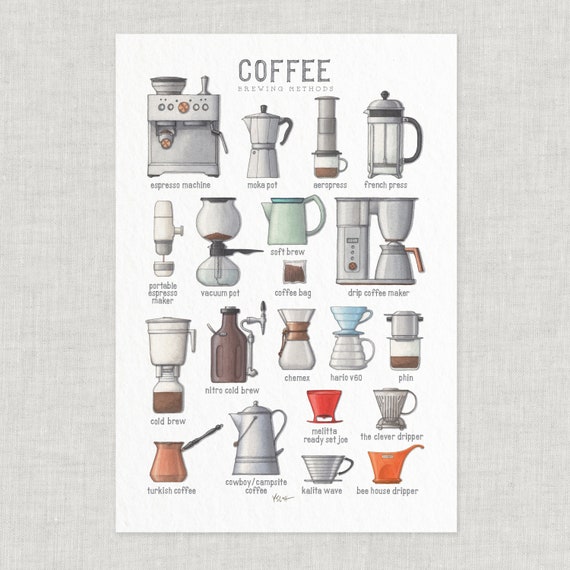The image is a rectangular poster entitled "Coffee Brewing Methods," showcasing a detailed array of approximately two dozen different coffee brewing devices against a light gray background. This highly informative poster features a mix of traditional and modern coffee-making techniques, each clearly labeled with descriptive text. The devices arranged from the upper left to the right and then downward include an espresso machine, mocha pot, AeroPress, French Press, portable espresso maker, vacuum pot, soft brew coffee bag, drip coffee maker, cold brew, nitro cold brew, Chemex, Hario V60, Fin, Melitta Ready Set Joe, The Clever Dripper, Turkish Coffee, Cowboy Campsite Coffee, K-Lite Wave, and Bee House Dripper. The visuals of these coffee makers, each meticulously illustrated, possess a faded color scheme, evoking a vintage, old-fashioned aesthetic.